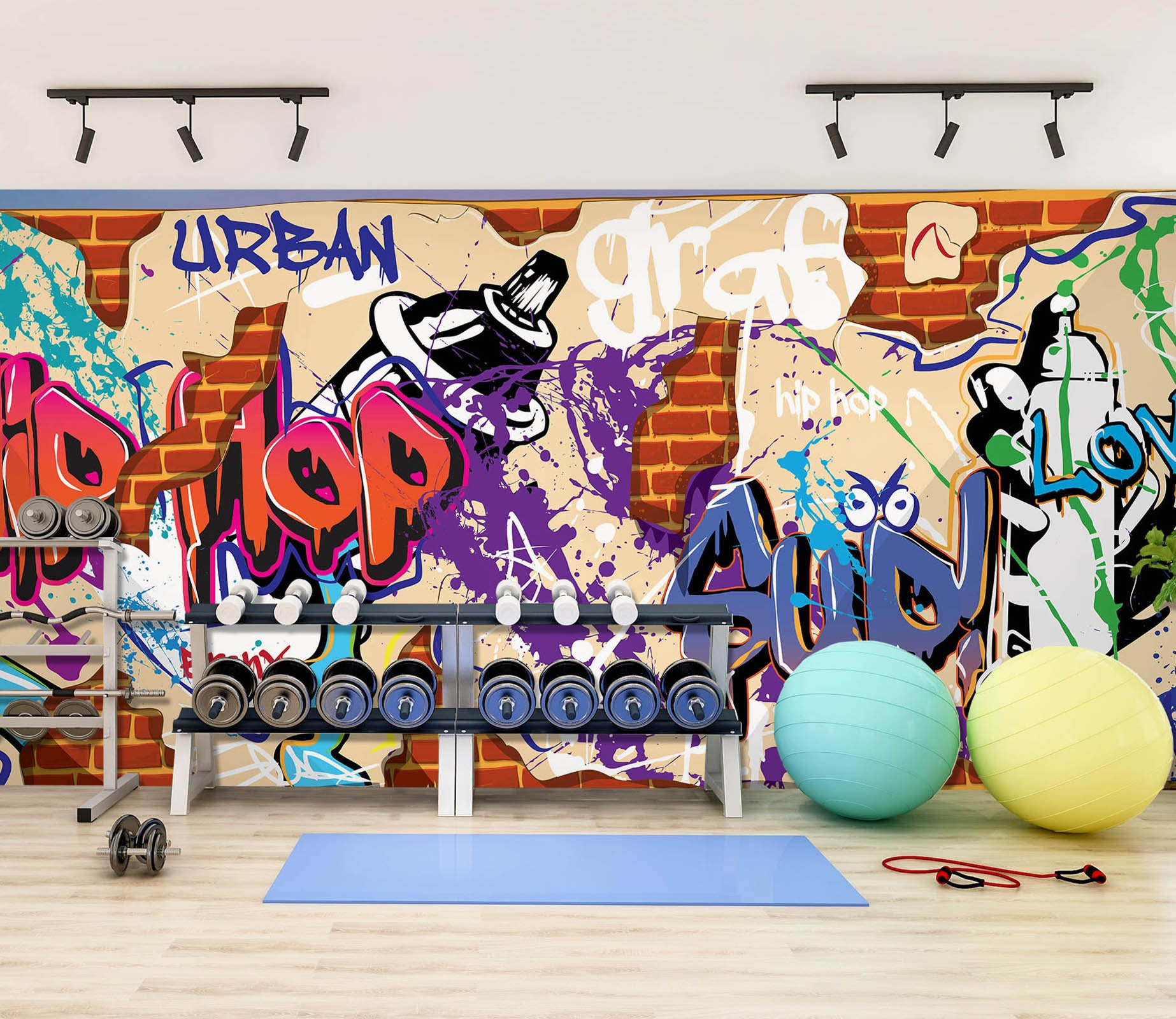The image showcases a vibrant gym interior, dominated by an urban graffiti wall teeming with splashy colors and a prominent spray paint can drawing. The off-white laminate wood floor contrasts with an upper beige section of the wall, highlighted by black spotlights. In front of the wall, a blue yoga mat is laid out on the floor, situated centrally with a set of dumbbells lying to its left. On the right, a mint green exercise ball and a golden yellow exercise ball lean against the wall, accompanied by a red resistance band. The gym's weight equipment includes a weight rack behind the yoga mat featuring individually shelved dumbbells and a secondary rack that partially visible, holding various bars used for bench press and curling exercises. The graffiti wall's artwork includes bold blue capital letters spelling "URBAN" at the top left, with the rest of the art featuring a dynamic mix of graffiti-style writings and vibrant, splashy colors that evoke the texture of reddish-orange bricks.